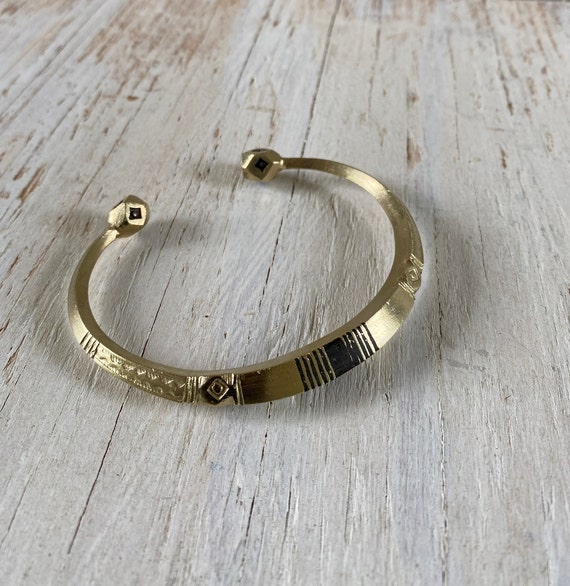The image features a finely detailed, gold, horseshoe-shaped ring placed on a backdrop of rustic, white antique-finished boards. The background, marked with numerous scratches and a light grayish beige tone with hints of brown, suggests an aged appearance, likely mimicking an old wooden floor or countertop. The ring, slightly more than a semicircle with an opening where two knobs do not connect, exhibits a thick to tapered design. Prominent details include black notches in the center, a small black, diamond-shaped eye to the left of the notches, and a gold, diamond-shaped eye to the right. To the left of the black eye is a section resembling a double-sided sawtooth blade, accompanied by additional small notches. The intricate markings and engraved designs lend the ring an ornate and elaborate look.